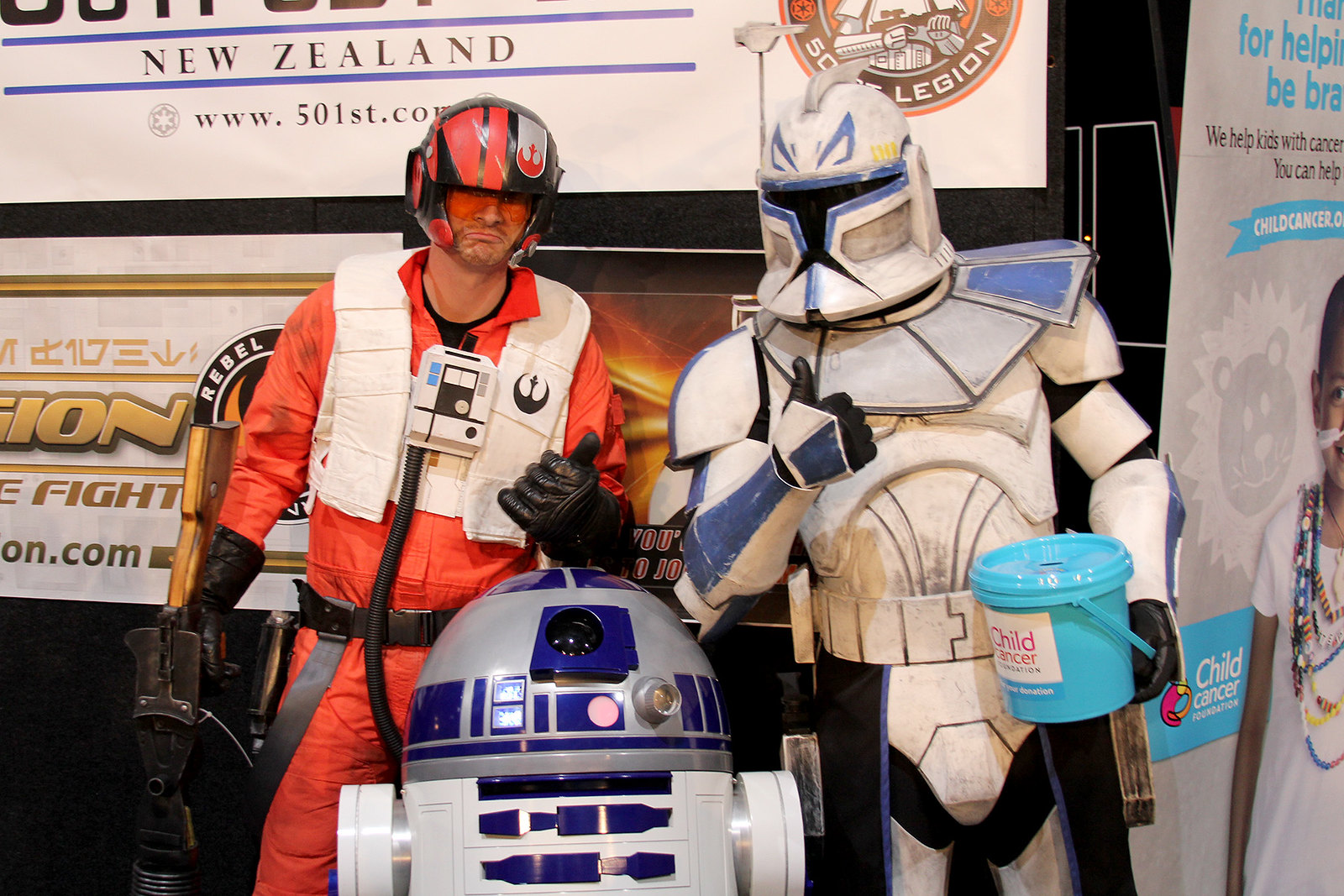In this detailed indoor photograph taken at a cosplay event or charitable convention dedicated to supporting children with cancer, we see two individuals dressed in distinct Star Wars costumes standing directly in the center of the image. The person on the left is adorned in an orange flight suit reminiscent of a Star Wars pilot, complete with a white vest, black hose, black gloves, and an orange helmet with red sections and goggles, wielding a black blaster weapon. Next to him, on the right, is another individual dressed as a stormtrooper in white armor with blue accents on the shoulders and helmet. This person holds a turquoise bucket marked for child cancer donations. Positioned between them is a life-sized R2-D2 statue featuring its iconic dome-shaped head and white and blue body. In the background, several banners and posters are visible with partial text including "New Zealand," "www.501st.com," and phrases such as "we help kids with cancer" alongside an image of a child's face. The colors in the image include white, blue, black, orange, red, yellow, tan, and gray, and the setting is clearly an organized indoor venue aimed at raising awareness and funds for children's cancer initiatives.